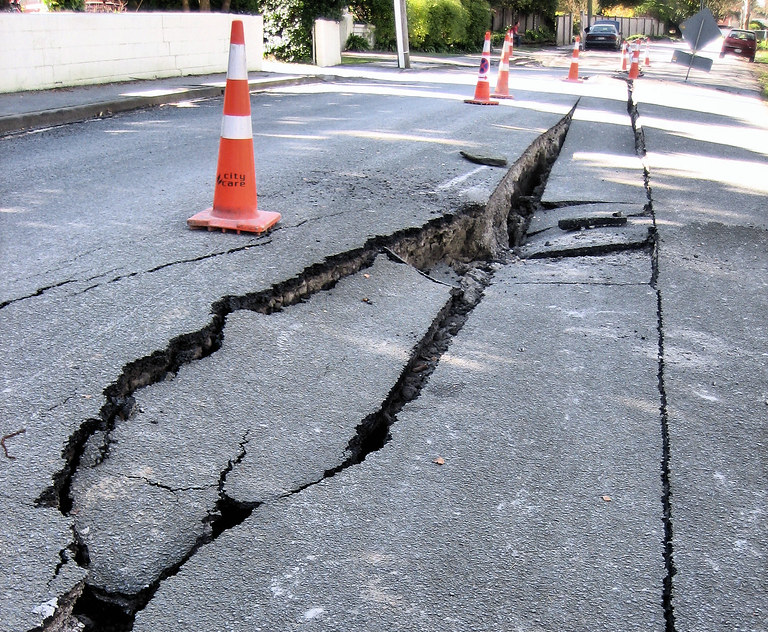The photograph illustrates a severely dilapidated street, riddled with large cracks, crevices, and potholes, suggesting significant damage, possibly due to an earthquake or another calamity. In the center, a substantial crack runs from left to right with indentations about six inches to a foot deep. Surrounding this damage, orange traffic cones with white stripes mark the area, indicating that the road is blocked for traffic. The dark grey, tarred pavement appears to be caving inwards, with sections missing. To the left side, a white concrete compound wall, likely enclosing another building, runs parallel to the sidewalk. At the top of the image, there is a gateway visible. Several cars are parked in the background on both sides of the road: a maroon car on the right-hand side and a dark black car to the left. Additionally, grey road signs are present, possibly warning incoming traffic to avoid this damaged section. The outdoor scene is clearly in need of repair work, with the cones and damage prominently emphasizing the road's hazardous condition.